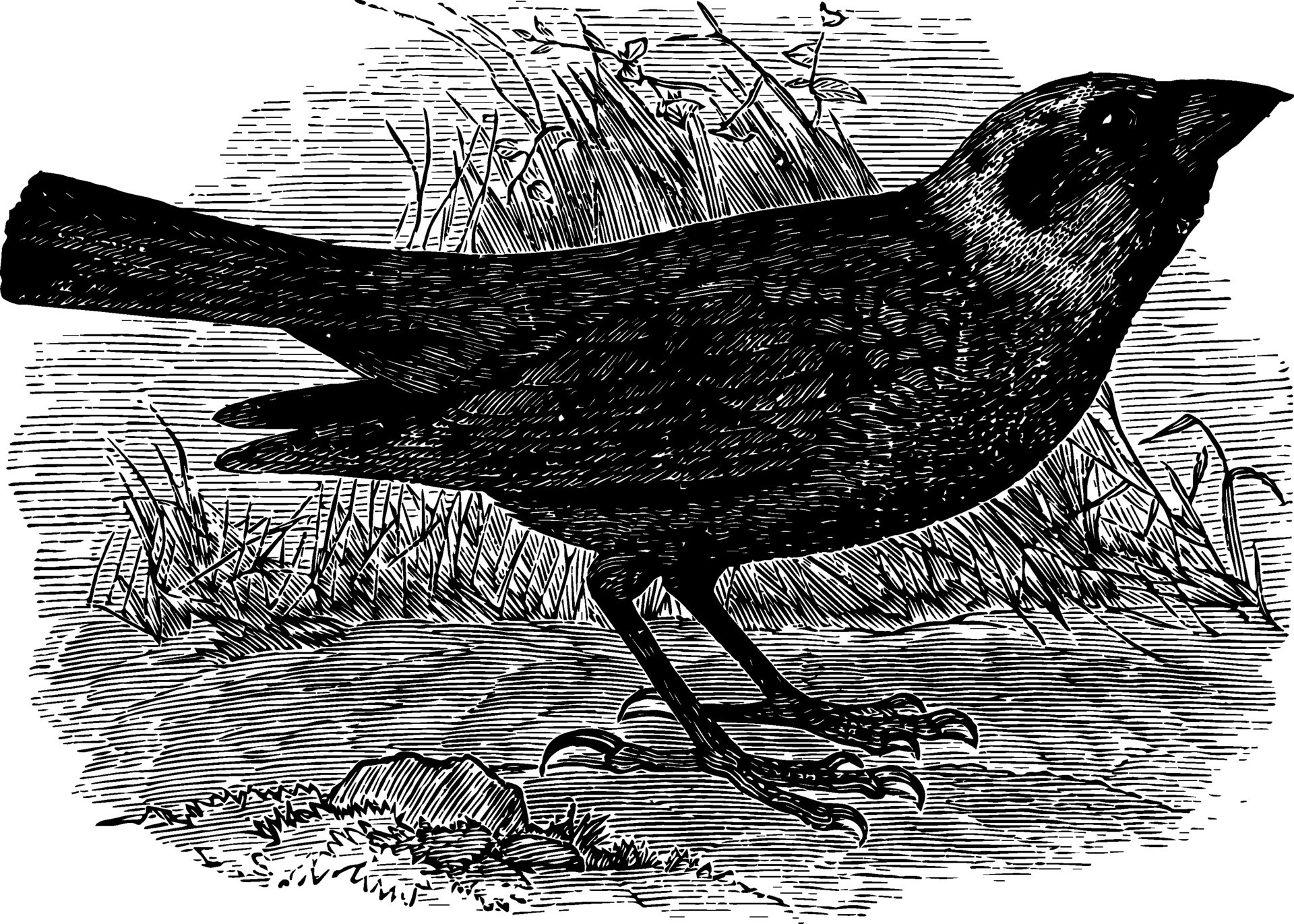This is a detailed black-and-white line drawing, reminiscent of early 1900s to 1920s etched block-style illustrations. The image features a black bird, specifically a crow or raven, rendered in a side profile as it looks upwards. The bird has black feathers, dark eyes, and distinctive pointy bird feet with three frontal toes and one rear toe, each digit adorned with long nails. Its wings are closed as it stands on intricately textured ground, characterized by fine hatching and cross-hatching techniques typical of the era. Surrounding the crow are various elements: in the background, there's a pile of straw or weeds, adding depth to the composition. Closer to the viewer’s perspective, in front of the bird, there is grass and a rock also detailed with hatching for shading, enhancing the graphic element of the illustration. The overall scene blends intricate pen work with a strong contrast, emphasizing the dark form of the crow against the relatively lighter background.